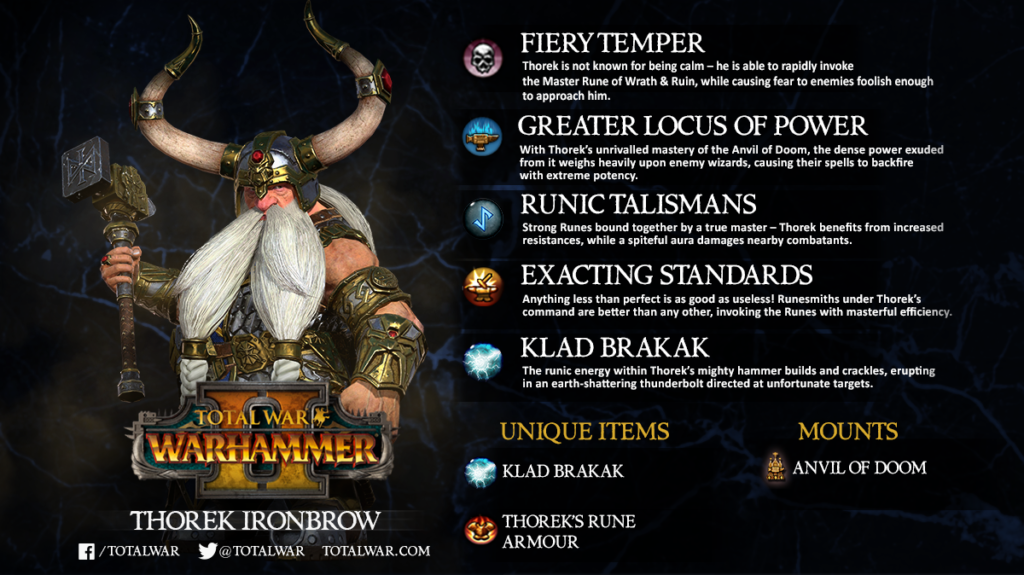The image is a horizontally-oriented advertisement with a black background, likely for a game or book cover titled "Total War Warhammer." On the left side, there is a detailed drawing of a character labeled in gold letters at the bottom as "Thorac Iron Brow." Above the name, it prominently displays "Total War Warhammer." The character is a warrior wearing an imposing helmet adorned with large horns and has a massive white beard divided into two ponytails. He also appears to be holding a big hammer and is clad in heavy armor. Below the character, there are social media handles for Facebook and Twitter, as well as a web address, TotalWar.com. The right side of the image lists attributes and descriptions of the character: "Fiery Temper," "Great Locus of Power," "Runic Talismans," "Exacting Standards," and "Clad Bracock," each with further elaboration underneath.